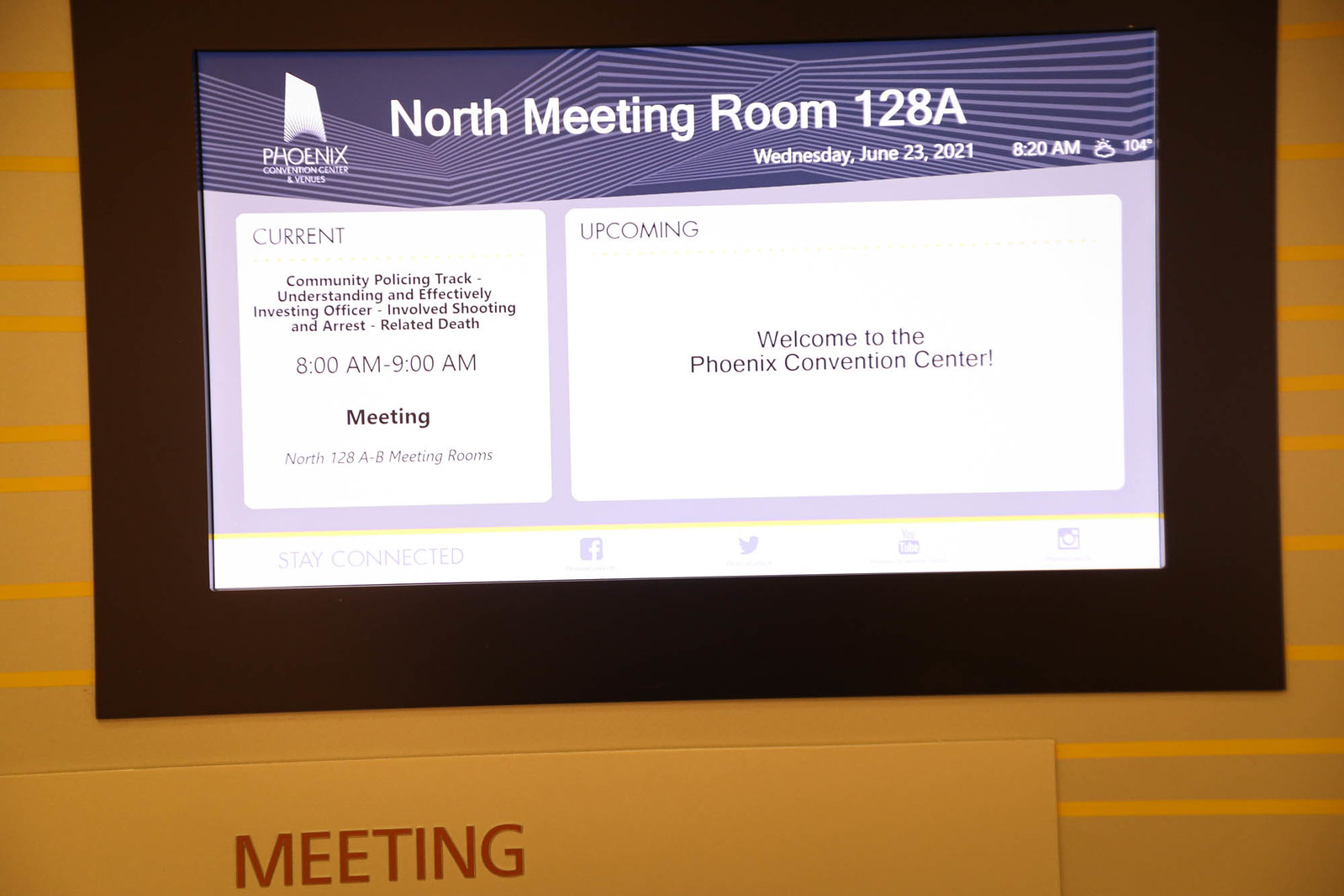The image depicts an indoor setting with a multi-colored patterned wallpaper in the background. Prominently featured towards the top is a television screen mounted on the wall, with a thick black border. The screen displays detailed event information for the Phoenix Convention Center and Venues. Specifically, it mentions North Meeting Room 128A, scheduled for Wednesday, June 23rd, 2021, at 8:20 a.m. The content on the screen indicates ongoing and upcoming sessions, with the current community policing track discussing topics such as 'Understanding Effectively Investing Officer Involves Shooting and Arrest-Related Death', running from 8 a.m. to 9 p.m. On the left side of the screen, the session is described in detail, whereas the right side highlights an upcoming event. At the bottom of the screen, there is a banner that includes the word 'Meeting' in red text. Additionally, in the bottom left corner of the image, there's a small poster that also reads 'Meeting'. The setting appears to be a meeting room at the Phoenix Convention Center, but it is unclear what time of day it is. The colors visible in the image are a mix of tan, yellow, black, dark blue, light blue, purple, and yellow.